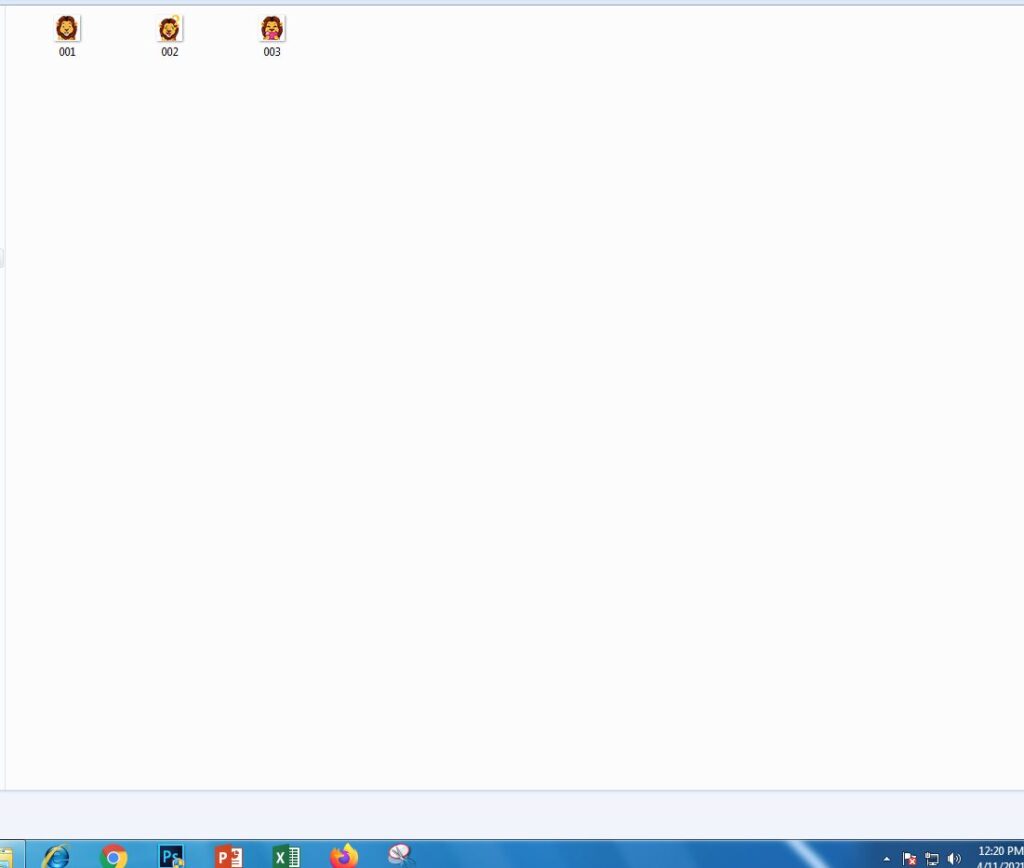The image is a screenshot taken from a computer screen, likely a laptop. The majority of the screenshot is dominated by a white background or a white box. At the bottom of the screenshot, the blue taskbar stretches across the screen, populated with various icons. From left to right, the icons include Internet Explorer, Chrome, and possibly applications like Publisher, Excel, and Firefox, with some being unidentifiable. 

On the far right side of the taskbar, the system clock is visible, displaying the time as approximately 12:20 p.m., though the date beneath it is cut off. Adjacent to the clock are familiar system icons such as volume control and network connection status.

In the main body of the image, there are three file thumbnails aligned vertically, each featuring a similar, indistinct image that might depict an animal. The filenames for these images are simply labeled "001," "002," and "003."